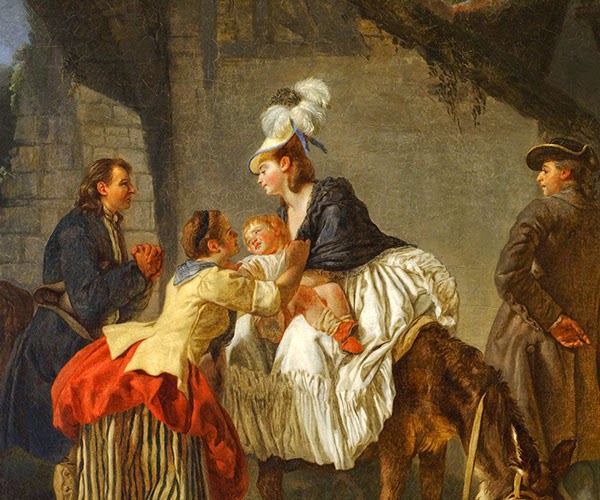In this detailed painting set in an old colonial era, four central figures are depicted against a backdrop of unadorned walls or stonework. On the left-hand side stands a man with shoulder-length hair, wearing a blue jacket and a gray belt. He holds a hat between his side and elbow in a pleading motion. To his right, a woman with a black headband, a blue scarf, and a yellow coat with white cuffs and a red petticoat is receiving a child from another woman. This child, with blonde hair and orange shoes, is being handed over by a woman seated on a donkey. The seated woman has brown hair and wears a black shawl, a white colonial skirt, and a hat adorned with feathers and a blue bow. On the far right, another man dressed in a gray-brownish long coat and a black colonial hat gazes at the scene, his hand resting behind his back. The overall composition captures a moment of delicate interaction and diverse attire typical of the colonial period, adding depth and historical context to the vibrant tableau.